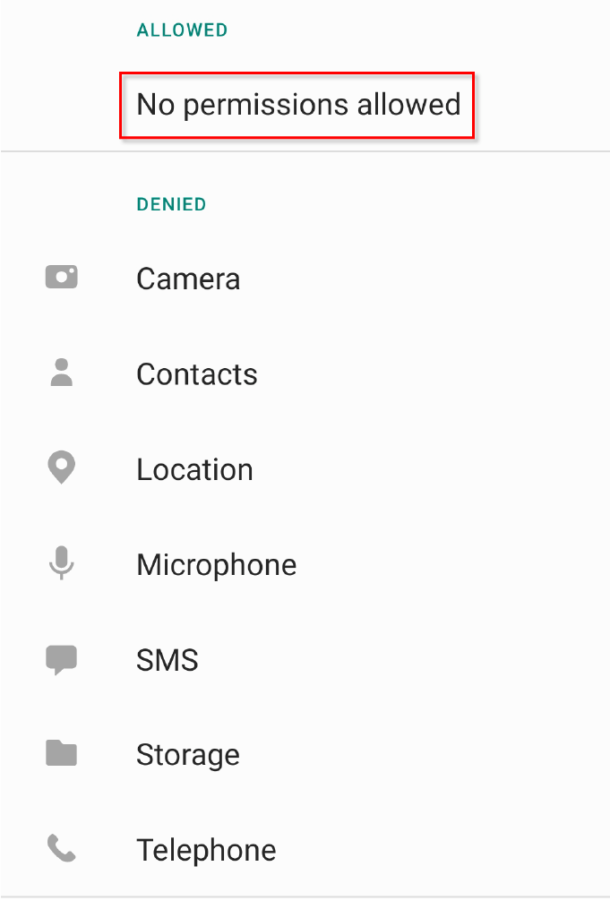**Caption:**

The image depicts a screenshot of a permissions settings screen, featuring a pale off-white background. At the top of the screen, the word "Allowed" is displayed prominently in blue text. Directly underneath, a rectangular box outlined in red with the phrase "No Permissions Allowed" is visible, indicating restricted access. Below this, the word "Denied" is written in green, signaling permissions that have been refused. 

Continuing down the screen, a list of icons paired with their respective categories of permissions appears. The sequence of icons and labels includes: a camera icon followed by the label "Camera," a contacts icon labeled "Contacts," a location icon followed by "Location," a microphone icon labeled "Microphone," an SMS icon next to "SMS," a storage icon paired with "Storage," and, lastly, a telephone icon accompanied by the label "Telephone." Each permission category is visually aligned to display the icon on the left and the corresponding name on the right.